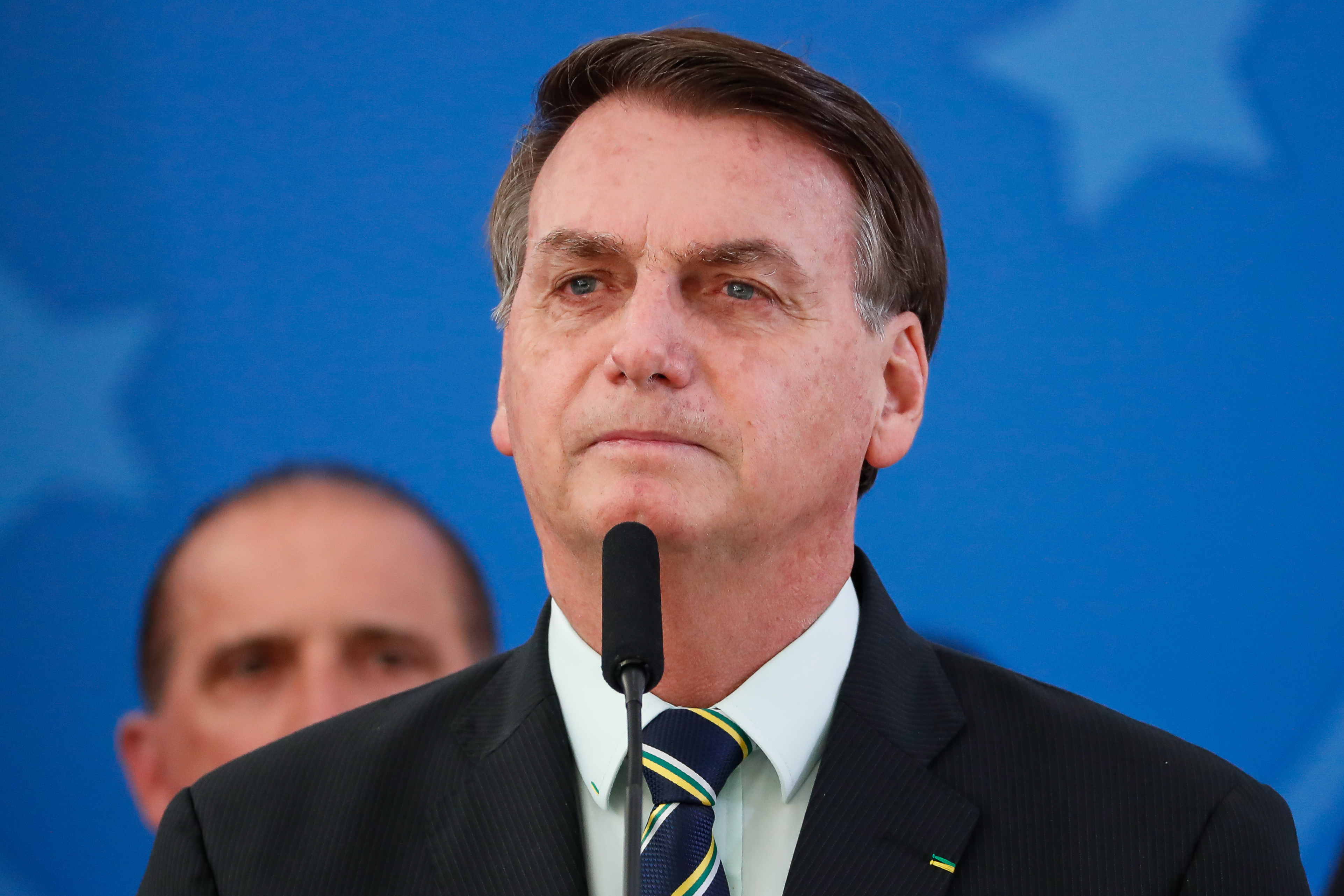This photograph captures former Brazilian president Jair Bolsonaro standing in front of a microphone, possibly delivering a speech or answering a question. He is dressed in a dark suit, specifically a black or dark blue jacket, paired with a white shirt and a blue tie adorned with yellow, blue, and white stripes, potentially reflecting the colors of the Brazilian flag. His brown hair, displaying hints of gray, is neatly parted to the side. A small, unidentifiable pin is visible on his left lapel. Behind Bolsonaro, slightly obscured by his right shoulder, stands another man with short hair, whose face is partially hidden, only his eyes are in view. The backdrop features a blue banner embellished with light blue or white stars, adding a formal and possibly patriotic atmosphere to the scene.